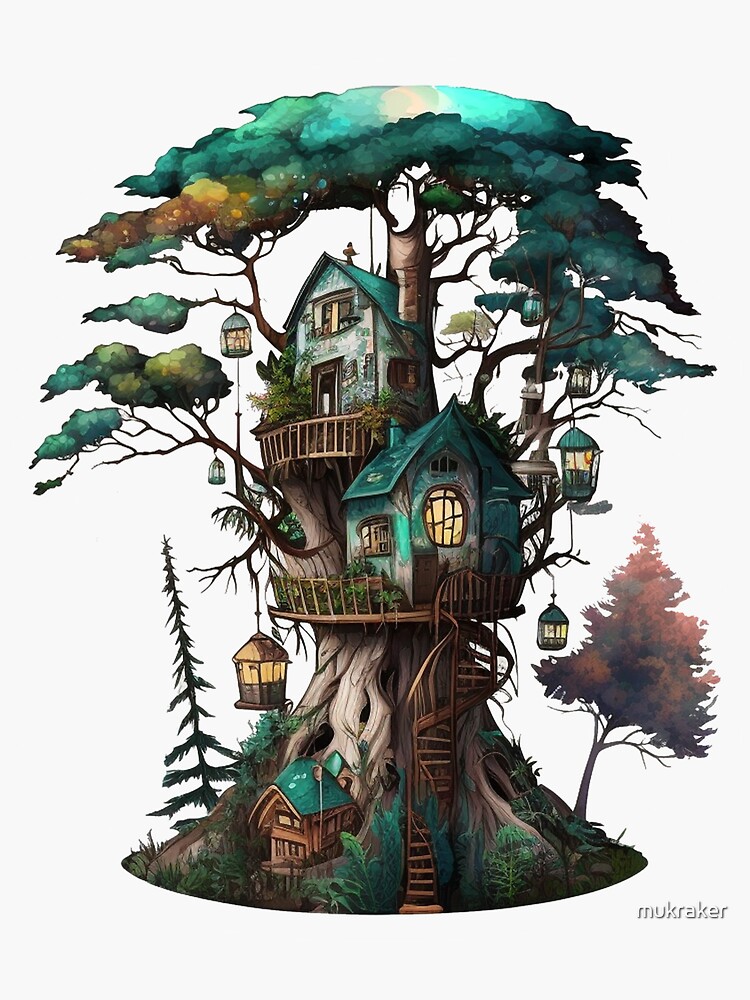Illustrated against a white background, this fantasy treehouse is drawn with exquisite detail, capturing a whimsical and magical essence. The tree is robust, with strong roots anchoring it firmly, and its trunk extends high, supporting a series of charming green houses. At the base of the tree, a small house sits, and a spiral staircase wraps sinuously around the trunk, leading to a medium-sized house in the middle, each with its own little porch and banister. Further up, near the top, another house perches beneath a canopy that envelops the scene, sprinkled with blue, gold, and teal leaves shifting towards autumn hues of orange and red.

Scattered along the branches are smaller houses, possibly birdhouses, adding to the intricate fantasy elements of the scene. Lanterns dangle from the branches, their soft light enhancing the magical atmosphere of the illustration. The artwork, presumably created by an artist named Muckraker, showcases an imaginative, storybook-like environment that is both enchanting and detailed.